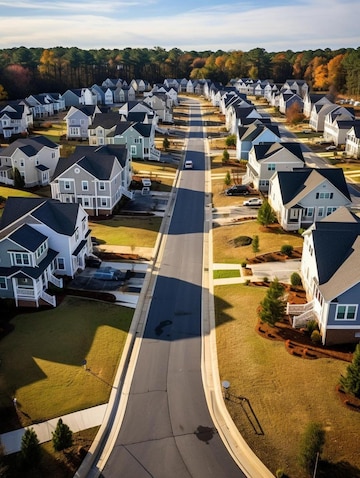This aerial photograph captures a meticulously organized suburban housing development set amidst a beautifully forested area during the fall. The neighborhood consists of neat rows of quadplex homes, each adorned with light gray walls, white accents, and navy blue slanted roofs. The houses are uniformly two stories high with a squared shape and white-framed windows. A gray paved road runs centrally through the image, bordered by light gray curbs and manicured green lawns.

At the top of the image, a thin strip of blue sky fades into a layer of clouds, casting a serene backdrop against the colorful forest below. The forest trees are in the midst of their autumn transformation, showcasing a palette of green, gold, and red leaves. The shadows cast by the houses suggest the photograph was taken on a mostly sunny day, likely in the evening. The yards are meticulously maintained with a yellowish-green hue, adding to the picturesque quality of the scene. Despite the perfect alignment and uniformity of the homes, the photograph hints at the possibility of AI generation due to its impeccable organization and design.